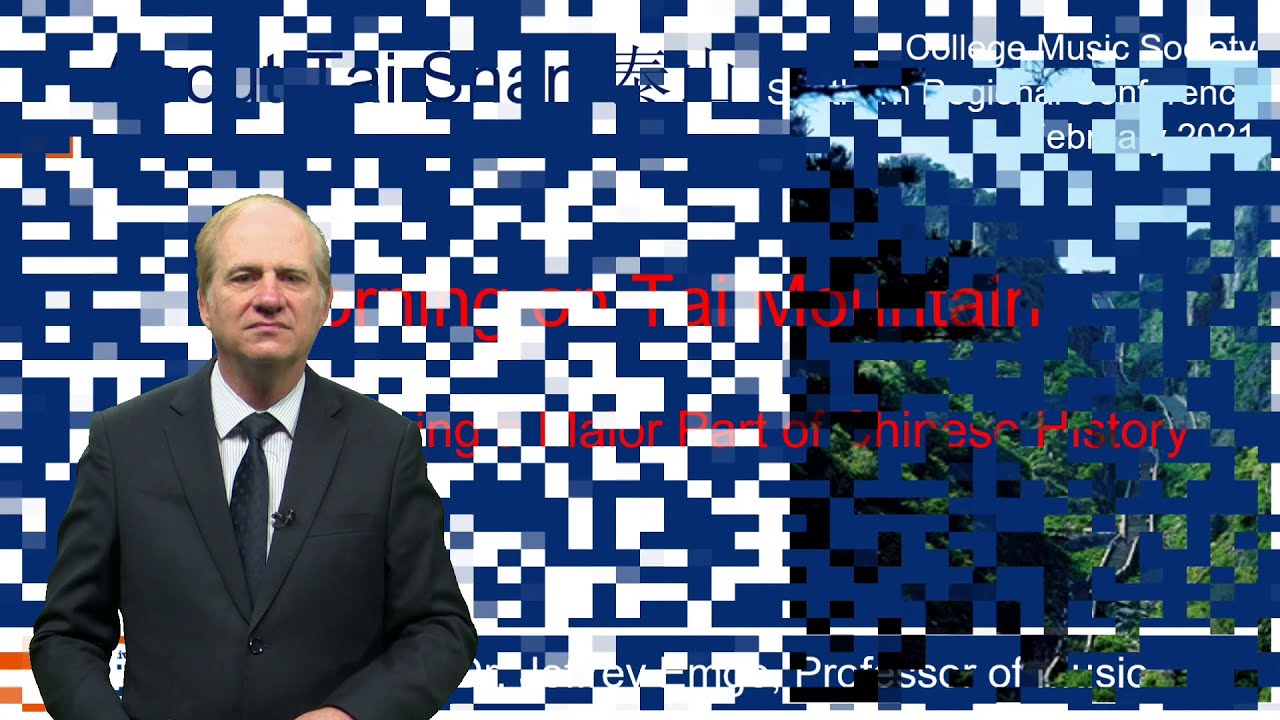The image displays an older Caucasian man, likely in his 50s or early 60s, standing in a predominantly blue and white, digitized background that resembles a partially formed digital scene. The man, positioned on the left side of the image, is wearing a gray or slightly bluish-gray suit with a dark navy tie and a white shirt. He appears to have thin white hair on the sides and a bald top, coupled with a larger nose and a frowning expression. The background is marked by pixelated blue, white, green, and black patterns, containing fragmented and overlapping text. Notable legible portions include "College Music" in the upper right, "professor of music" in the bottom right, and isolated red words like "mountain" and "history." The overall scene suggests an incomplete or transitioning screen, possibly indicative of a paused or glitching digital media such as a podcast recording.